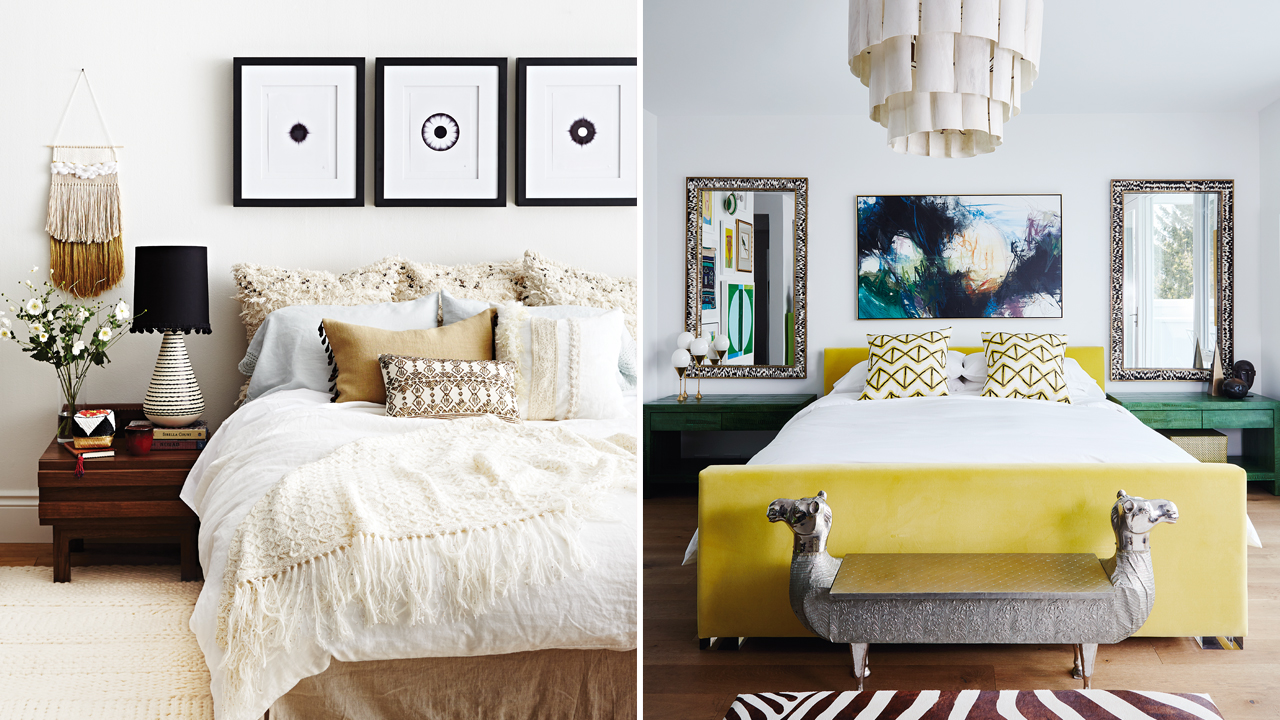The image is a collage of two bedrooms side-by-side, each with distinct styles and elements. 

On the left side, the bedroom features a serene Scandinavian-inspired design. The walls are painted white, adorned with three simple black-framed circular designs above the bed. The bed itself is dressed in white linens and a light tan bedspread, accented by multiple pillows in shades of white and brown. A soft white throw blanket adds extra coziness. Below the bed, there's a white throw rug laid on a hardwood floor. To the side, a brown end table supports a white lamp with a black cone-shaped lampshade. Decorative touches include a small vase of flowers and hanging ornamental art resembling a skirt.

On the right side, the bedroom exudes a modern contemporary feel with a touch of glamour. Central to the design is a bed with a striking yellow velvet headboard and base. The bed is made with crisp white sheets and is accented by patterned yellow and white pillows. Flanking the bed are two green nightstands, each topped with intricate mirrors framed in what appears to be silver sparkle. A striking abstract painting with multiple colors, including red, blue, black, and purple, hangs above the bed. The room features a brown hardwood floor with a zebra print rug in front of the bed, where a unique camel-head bench stands out as an eye-catching element. A white chandelier adds an elegant finishing touch to the space.